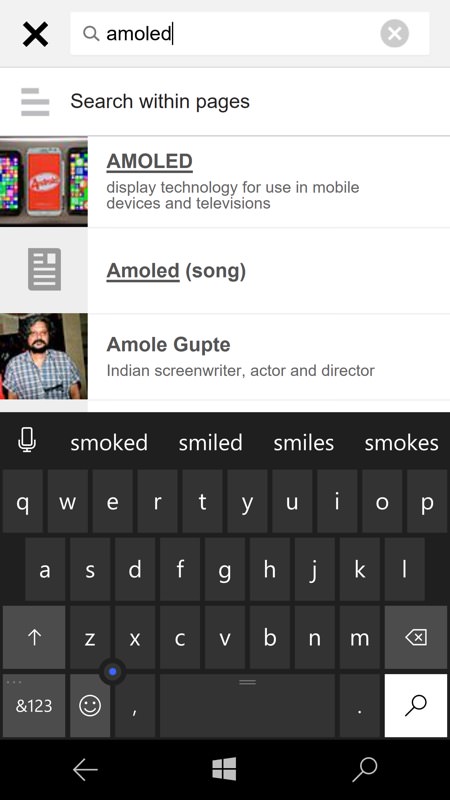The image depicts a high-resolution AMOLED display highlighted with various interface elements and text details. At the top of the screen, there is a grey bar featuring an 'X' symbol on the left. Below this, the word "AMOLED" is prominently displayed in large text. 

A closer view reveals a grey square icon resembling a document page, captioned "AMOLED (song)." An individual with curly hair and a thick beard is also shown, wearing a flannel shirt with a combination of blue and either yellow or white colors. The text next to this person identifies them as an "Indian screenwriter, actor, and director."

Further down, a virtual QWERTY keyboard is visible with text prediction suggestions such as "smoked," "smiled," "smile," and "smokes." Above the keyboard, navigation elements include a left arrow, a symbol resembling Microsoft's logo, and a magnifying glass icon, all set against a black bar. The top section of the display features a black square on a white background, with an additional grey bar at the very top. Overall, the image provides a comprehensive examination of AMOLED display technology and associated user interface components.